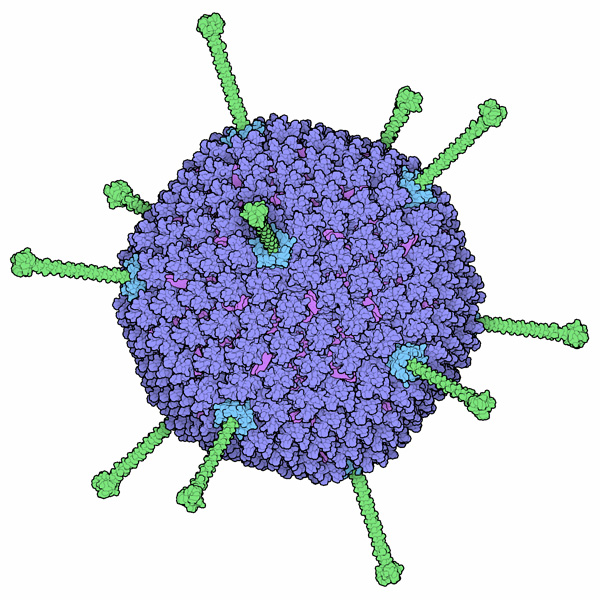This detailed, color illustration, rendered in a square format, depicts a spherical, computer-generated virus or microbial structure reminiscent of the COVID-19 virus. The main body of the illustration is predominantly blue, accentuated by light blue areas where green, spike-like protrusions emerge. These spikes, totaling approximately 11-12, extend outward in all directions and have a mint green hue with bulbous ends. Interspersed within the spherical form are areas of pink, adding to its intricate and textured appearance. The entire image sits against a stark white background, emphasizing the detailed, clustered, and fluffy texture of the virus-like structure.